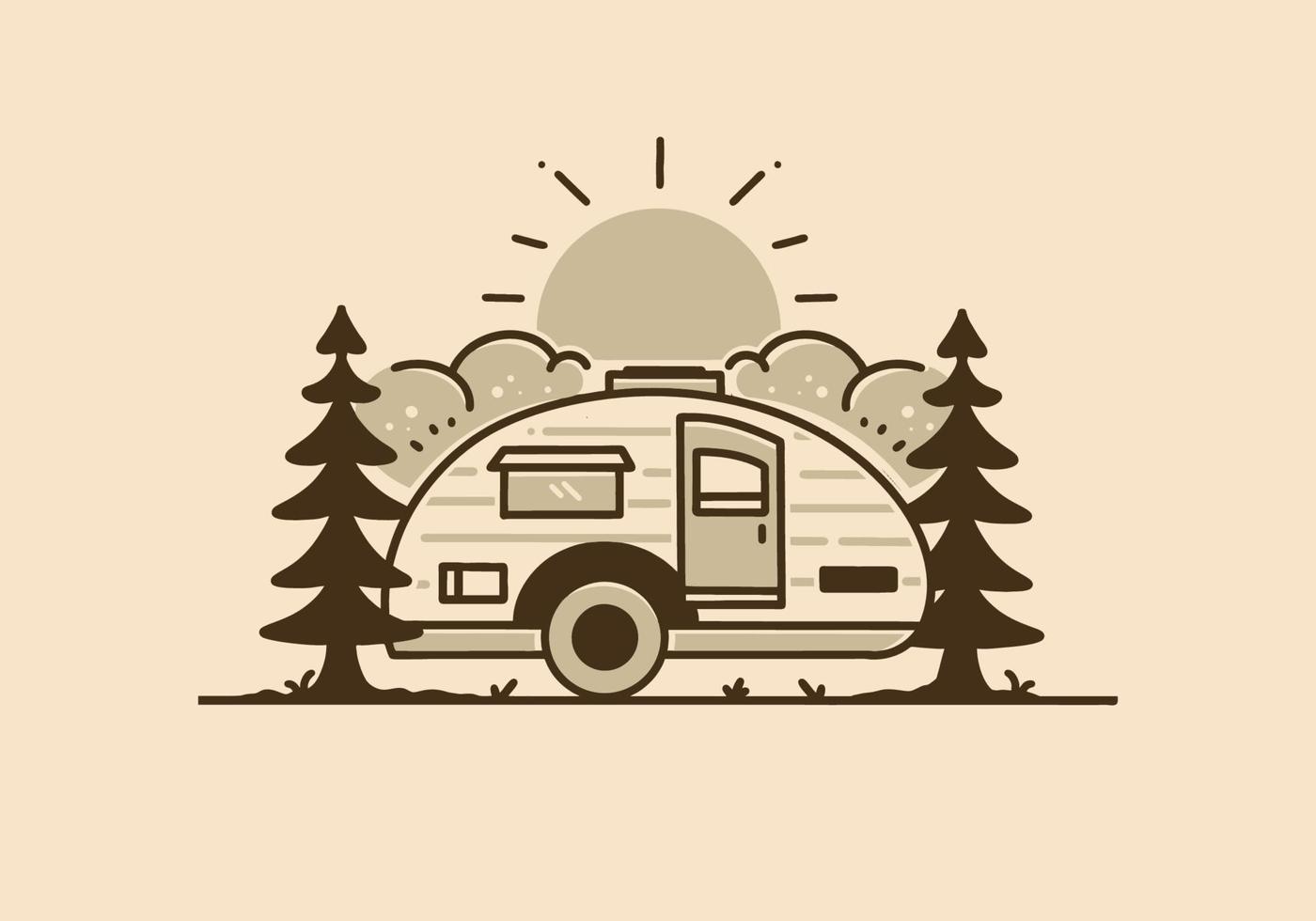In this rectangular illustration, rendered primarily in shades of gray and black against an off-white background, the focus is on a whimsically designed RV with a half-moon-shaped top and a single prominent wheel, positioned sideways. The RV features a detailed door and window, providing a sense of structure and livability. Flanking the RV on both sides are stylized black pine trees, enhancing a sense of natural surroundings. Above, centrally aligned, float several puffy clouds, their outlines neatly defined in black. Overseeing the entire scene from the center top of the image is a simple, radiant sun, depicted with clean lines that signify its rays extending outward. The composition blends elements of digital art and cartoon-like charm, creating an engaging and imaginative visual narrative.